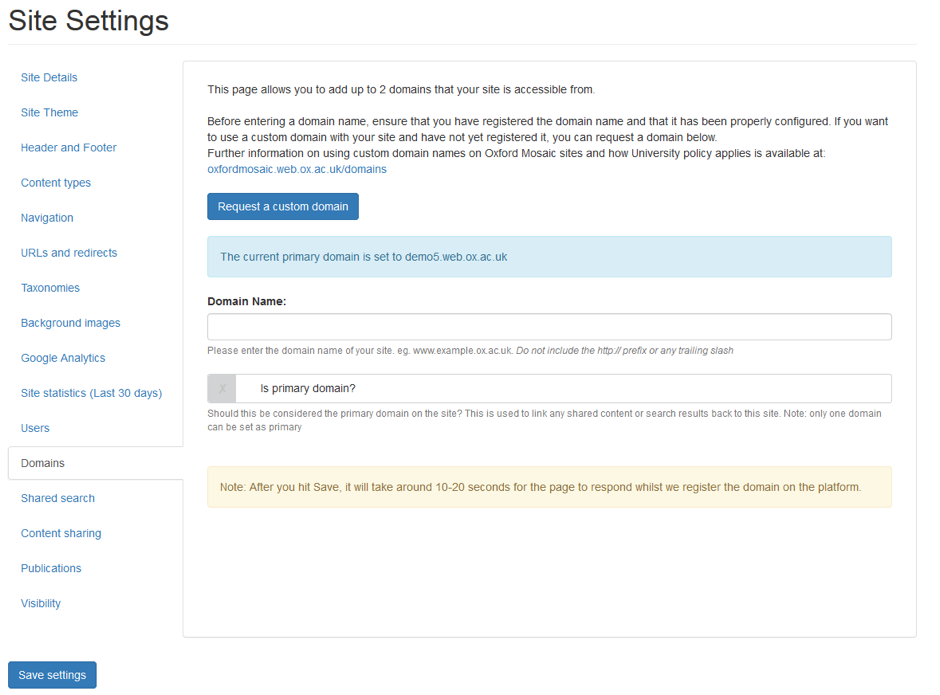This image is a detailed screenshot of a computerized interface for managing website settings, specifically tailored for domain management. In the upper left corner, the heading "Site Settings" is visibly prominent, setting the context for the page's function. Below the heading, a vertical navigation menu is featured, with clickable blue links labeled: "Site Details," "Site Theme," "Header and Footer," "Content Types," "Navigation," "URLs and Redirects," "Taxonomies," "Background Images," "Google Analytics," "Site Statistics," and "Users."

Adjacent to this menu, the main content area of the screenshot displays a bordered rectangular section. This section provides functionalities for domain configuration. At the top, an informative message indicates, "This page allows you to add up to two domains that your site is accessible from," alongside a thorough description.

Central to this section is a prominent blue button labeled "Request a Custom Domain." Below the button, a light blue horizontal bar spans the width of the rectangle, with the current primary domain specified as "demo5.web.ox.ac.uk."

Beneath this, there are input fields for domain configuration. The first labeled field titled "Domain Name" instructs users to "Please enter the domain name of your site." Directly below, a checkbox query labeled "Is Primary Domain?" is accompanied by a question mark icon for additional information.

At the very bottom of this section, a wide yellow horizontal bar issues a critical note: "Note, after you hit save, it will take around 10 to 20 seconds for the page to respond whilst we register the domain on the platform."

Overall, this screenshot exemplifies a website management interface designed for adding and customizing domains, providing a user-friendly and detailed process for domain registration and management.